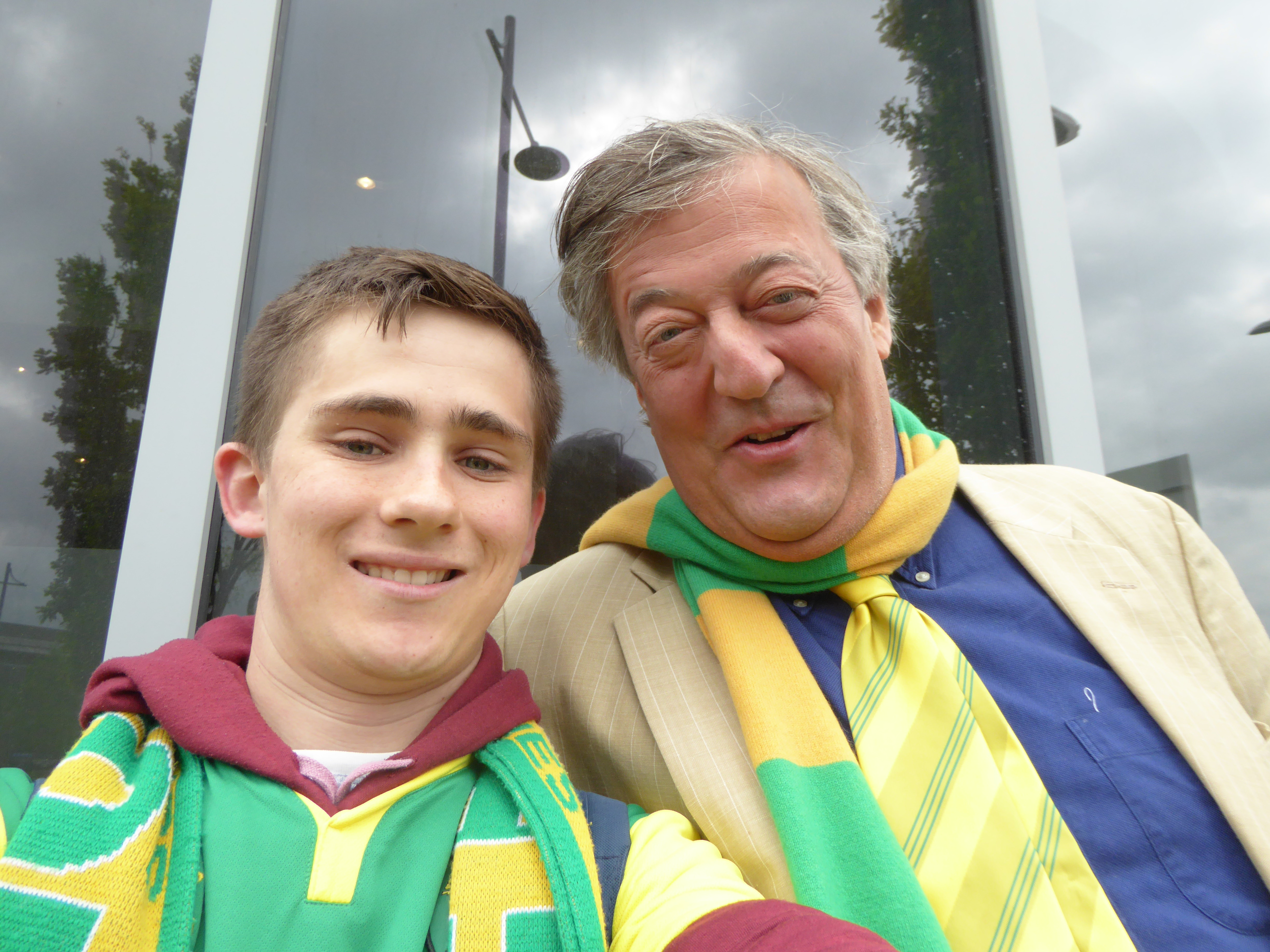In this close-up image, two males are positioned in the forefront, both smiling directly at the camera. On the left, a younger man, possibly a teenager or young adult, has brown hair and is donning a maroon-colored hoodie. Over his hoodie, he wears a green and yellow scarf, which gives the impression of a college accessory, coupled with a green shirt. To his right stands an older man, likely in his 50s, characterized by his gray hair and older facial features. He is dressed in a blue button-down shirt, adorned with a green and yellow striped tie, and a tan suit jacket with white pinstripes. Completing his attire is a matching green and yellow scarf. Behind them, glass windows or doors reflect the silhouettes of trees and a tall light post, adding depth to the scene.